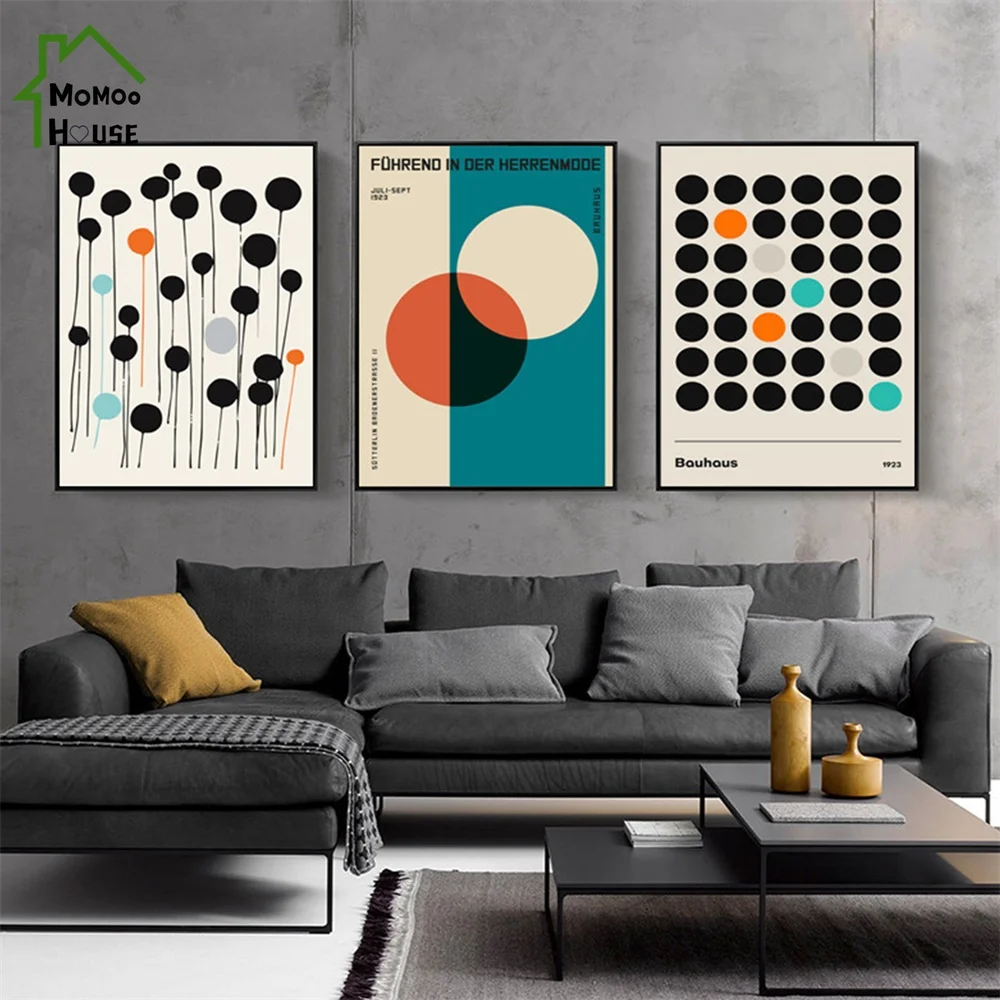This detailed photograph captures a modern living room, showcasing a large sectional dark gray couch adorned with several pillows in varying hues of gray and a notable bright yellow pillow on one end. A black and gray checkered blanket is casually draped over the far left side of the couch. 

In front of the sofa, there are two overlapping coffee tables—a shorter, modern black one layered beneath a taller, wooden one. These tables rest on a gray rug with dark fringes along the edges. Atop the coffee tables are yellow decorative items and some scattered papers. 

The gray wall behind the couch features three pieces of black-framed art. The left artwork consists of black and colorful circles with thin stems, resembling abstract balloons or flowers. The central piece, marked with German text, showcases a teal and white geometric design with overlapping circles in teal, orange, and black hues. The rightmost picture illustrates an abstract composition of predominantly black dots interspersed with occasional teal, orange, and blue dots, with "Bauhaus 1923" inscribed at the bottom.

In the top left corner of the photograph, a watermark is visible, displaying a green house outline enclosing the words "Moo Moo House." The second "O" in "House" is ingeniously replaced by a heart shape, emphasizing a playful and cozy atmosphere.